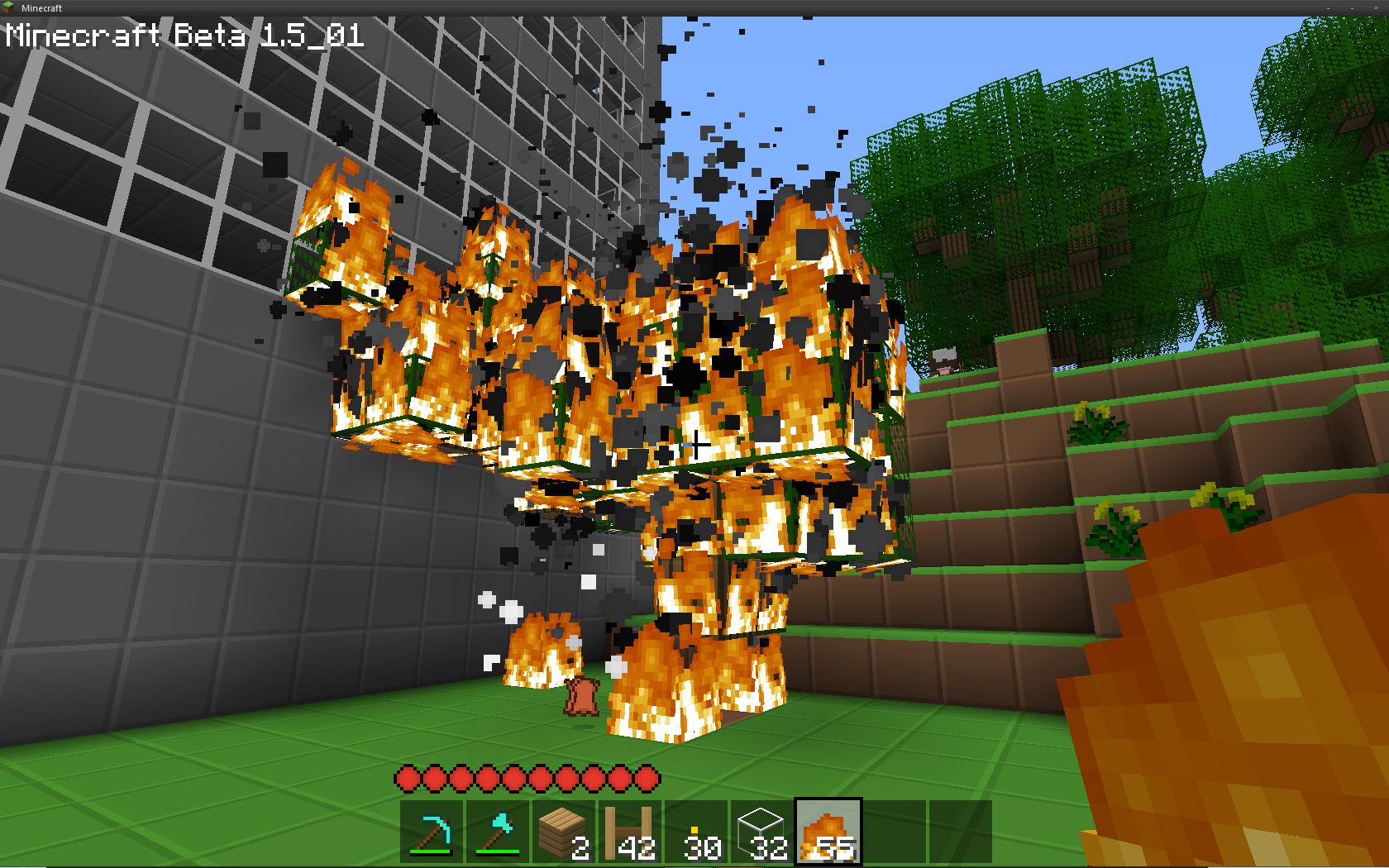This screenshot from Minecraft Beta 1.5.0.1 showcases a dramatic scene centered around a large structure made of blocks that are on fire. The structure stands atop a green ground, set against a background of tiered walls with a brown and lime color scheme, resembling planters with a few flowers. To the left, there is a gray building with darkened windows, while trees are visible on the right under a clear blue sky. The lower section of the screen displays the player's inventory, featuring items like a pickaxe, an axe, some boxes, potentially fences, as well as an undefined orange object in the bottom right corner.